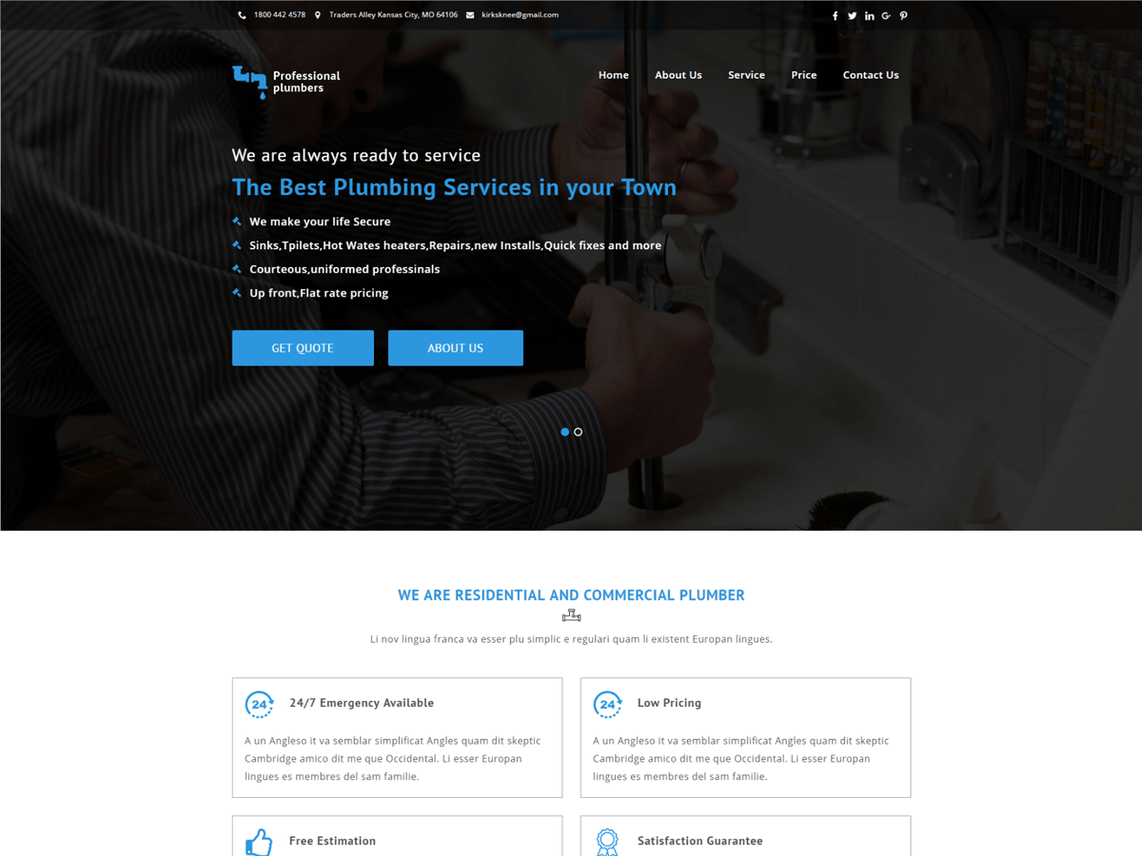This is a website for professional plumbers featuring a sleek black background with contrasting white and blue text. Subtly embedded in the background, a detailed image shows a person's hand gripping an object in a bathroom, likely a sink fixture. The individual is dressed in a long-sleeved, striped shirt. Prominently displayed in white text are the words "Professional Plumbers," followed by the reassuring statement, "We are always ready to service." Beneath that, a blue text section proclaims, "The best plumbing services in your town." Further down, four lines of white text offer additional information: 
1. “We make your life secure.”
2. "Sinks, toilets, hot water heaters, repairs, new installs, quick fixes, and more."
3. “Courteous, uniformed professionals.”
4. "Upfront flat rate pricing."

This comprehensive and visually appealing layout emphasizes the readiness, expertise, and customer-centric approach of the plumbing service.